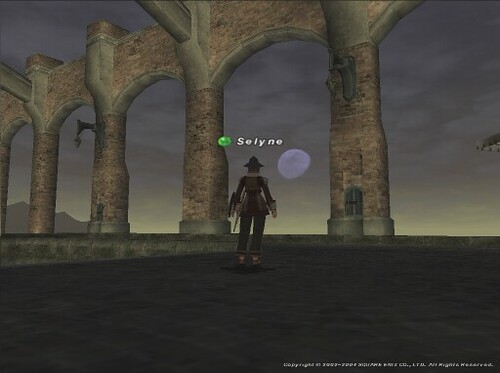The image, a still from a video game, captures an epic and foreboding scene featuring a character named Selene. Dominating the frame are monumental stone archways made of tan brown stone, stretching horizontally across the image. The ground beneath is made of a gray stone floor, adding to the ancient and atmospheric setting. In the middle of the image stands Selene, appearing to be a video game warrior from olden times. Selene is seen from behind, wearing a pointy hat with a brim and gauntlets. They seem to be holding a weapon, possibly a gun, in their left hand, and a sword is visible sheathed on their belt. Above their head, a lit-up moon is visible against a gray, foreboding sky that shifts to yellow near the horizon, suggesting a twilight atmosphere. The name "Selene" is prominently displayed above the character, indicating the player or character's name in the game. The intricate and grandiose architecture combined with the atmospheric lighting creates a sense of an epic quest underway.